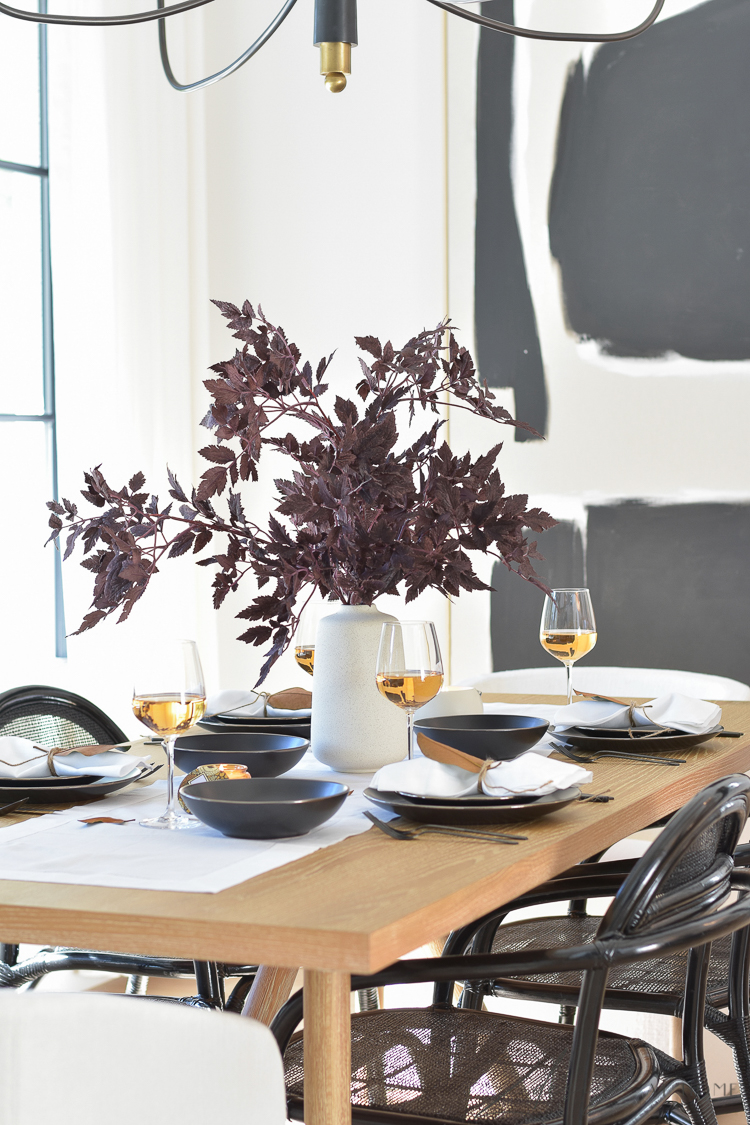The image depicts an elegant dining room that could either be in a very classy restaurant or a well-appointed home. The focal point is a light brown wooden table, adorned with a white runner down the middle. Around the table are four place settings consisting of dark slate gray plates and bowls, accompanied by silverware and white cloth napkins. Each setting includes a wine glass, about half-filled with a goldish liquid. Surrounding the table are four chairs, upholstered in a sleek gray tone. The table's centerpiece is a striking white vase filled with tall branches featuring purple leaves that spread wide across the tabletop.

The walls of the room are a soft, neutral shade of gray, with two large, modern, abstract paintings to the right. These artworks feature a white background with bold, dark gray strokes, creating a striking contrast. The overall ambiance of the room is sophisticated and inviting, blending contemporary art with classic dining décor.